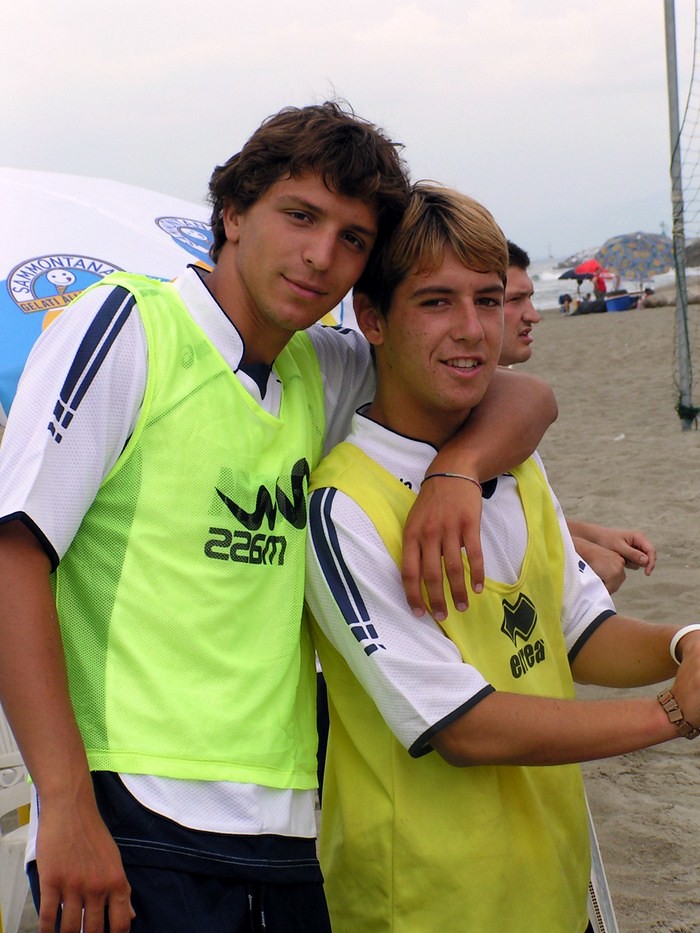The photograph portrays two young Caucasian men standing close together on a cloudy day at the beach, seemingly participating in a sporting event. Both men are wearing white jerseys covered by colored vests— the man on the left sports a green vest over his jersey, while the man on the right wears a yellow one. The man on the left, who is attired in blue shorts and a bracelet on his left arm, affectionately drapes his left arm around the shoulders of the man on the right. The man on the right is adorned with a white bracelet on his left arm and a wooden bracelet on his right arm. They stand in a slightly sideways position, facing the camera with serious expressions.

Behind the two men, a third man is visible in the background, looking away from the camera. The backdrop includes sand, beach umbrellas, and a small portion of a volleyball net to the right side of the image, enhancing the beach setting. Additionally, there’s a pole and a hint of a net visible, as well as a white and blue umbrella with the text "San Montana Gelati" and an image of a gelato cone. The sky is overcast with thick clouds, obscuring the sun. Some people can be seen laying on the sand under umbrellas, adding to the lively beach atmosphere.